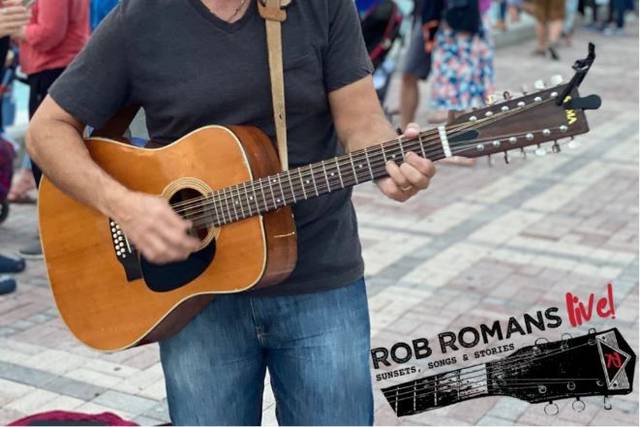The image captures a man playing a wooden 12-string steel guitar with a capo clipped onto the neck, though it is not currently in use. The man, dressed in a grey v-neck t-shirt and blue denim jeans, has the guitar strapped around his shoulder. The photo is framed from his shoulders down to his knees, so his face is not visible. The background depicts a bustling street with people standing and chatting on the sidewalk, slightly blurred to emphasize the musician. The setting appears to be outdoor, with ceramic tiles in shades of tan, dark green, and faint red underfoot. In the bottom right corner, a logo reads "Rob Roman's Live: Sunsets, Songs, and Stories," accompanied by the image of a guitar's top. The overall quality of the image is very good, highlighting the street performance ambiance.